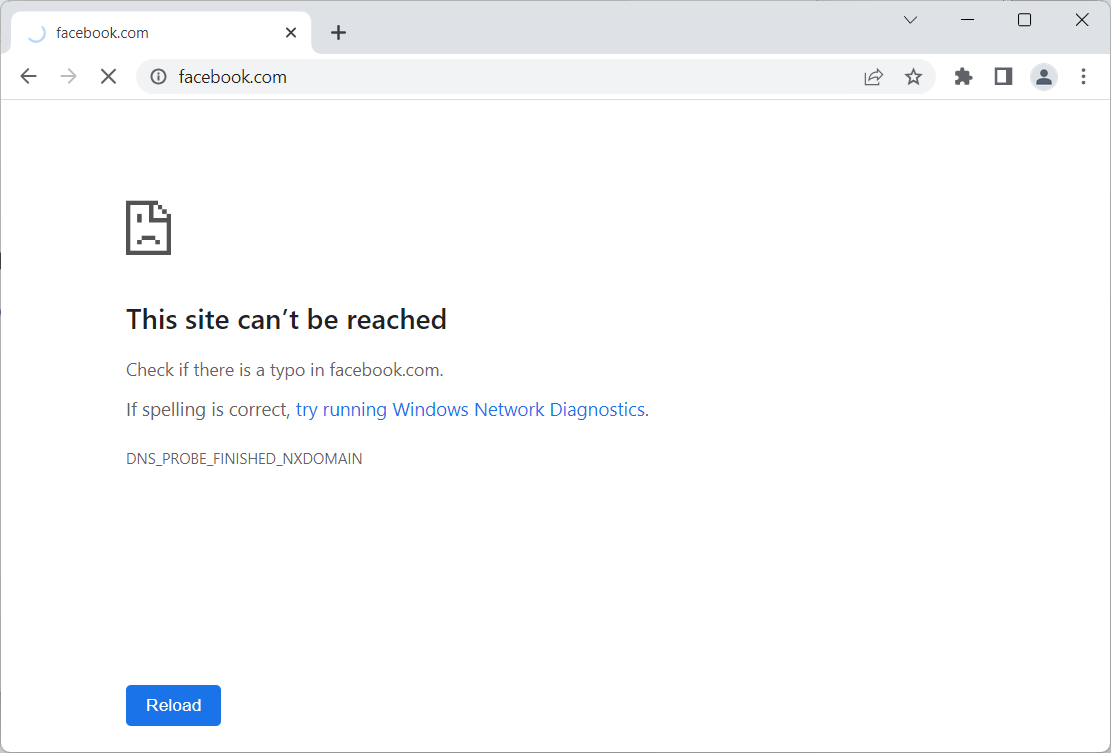A screenshot of a Facebook login attempt displays a browser window with a Facebook.com tab open, indicated by the tab visible in the upper left-hand corner. The tab shows a blue loading circle next to the text "Facebook.com." Next to it are navigation arrows (left and right), an 'X' button, and the URL "Facebook.com." In the top-right corner of the browser, there are control icons: a close button (X), a maximize/restore button (square), a minimize button (horizontal line), and a down arrow.

Beneath the URL bar, the webpage presents an error message predominantly against a white background. A small icon of a folded sheet of paper with a sad face is visible, symbolizing a page load error. Below this icon, bold black text states, "This site can’t be reached." In smaller, non-bold text, it suggests, "Check if there is a typo in Facebook.com.” The following line advises, “If spelling it correctly, try running Windows Network Diagnostics.” The error identification is stated as "DNS_PROBE_FINISHED_NXDOMAIN."

At the bottom of the error message, there is a blue button labeled "Reload" in white text, indicating an option to retry loading the page.